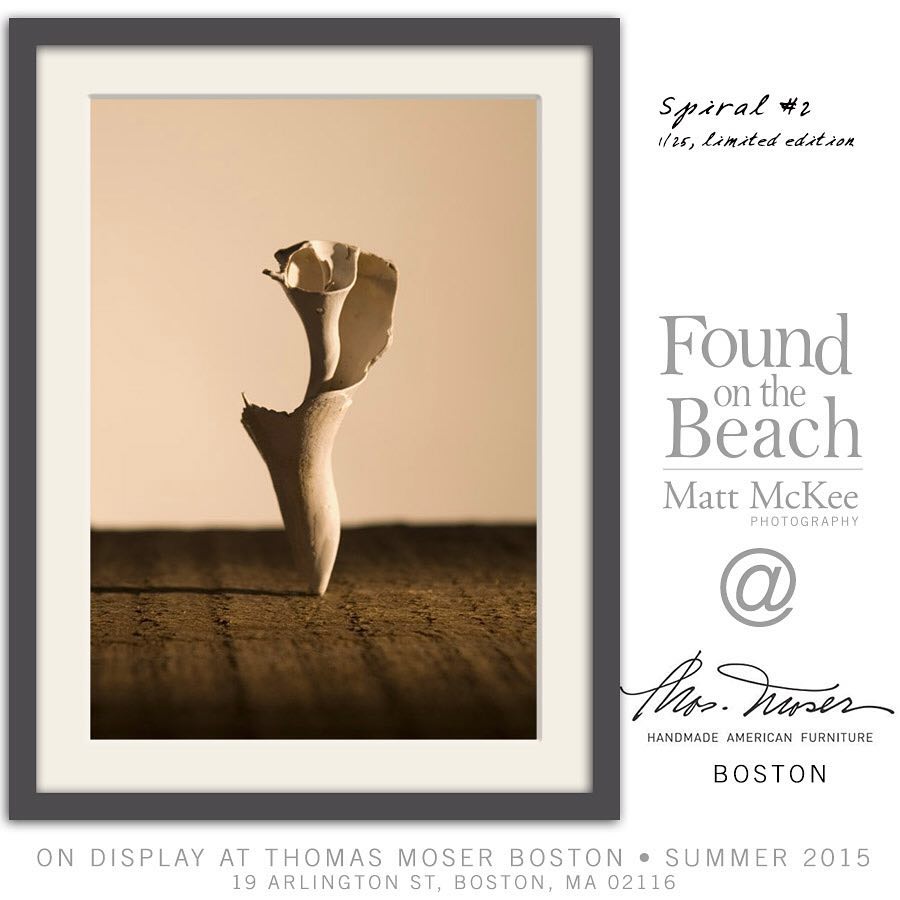This digital advertisement showcases a limited edition piece of art titled "Spiral No. 2," created and photographed by Matt McKee Photography. The photograph, displayed inside a white and gray frame, depicts an intriguing object that evokes the appearance of a conch shell or a spiral bone. It stands vertically on a meticulously detailed, dirt-like surface arranged in straight, perpendicular lines. The artwork, labeled as "1 of 25 Limited Edition," captures a phantasmagorical scene that could be described as resembling a wood shaving or a mushroom.

To the right of the image, there is text indicating that the artwork is part of the "Found on the Beach" photography series. This piece will be exclusively exhibited at the Thomas Moser Boston showroom, located at 19 Arlington Street, Boston, Massachusetts. The exhibit will be available for viewing only during the summer of 2015. Additionally, an emblem at the bottom signifies that the exhibit also emphasizes the theme of "Homemade American Furniture." This captivating and unique piece blends natural artistry with thoughtful presentation.